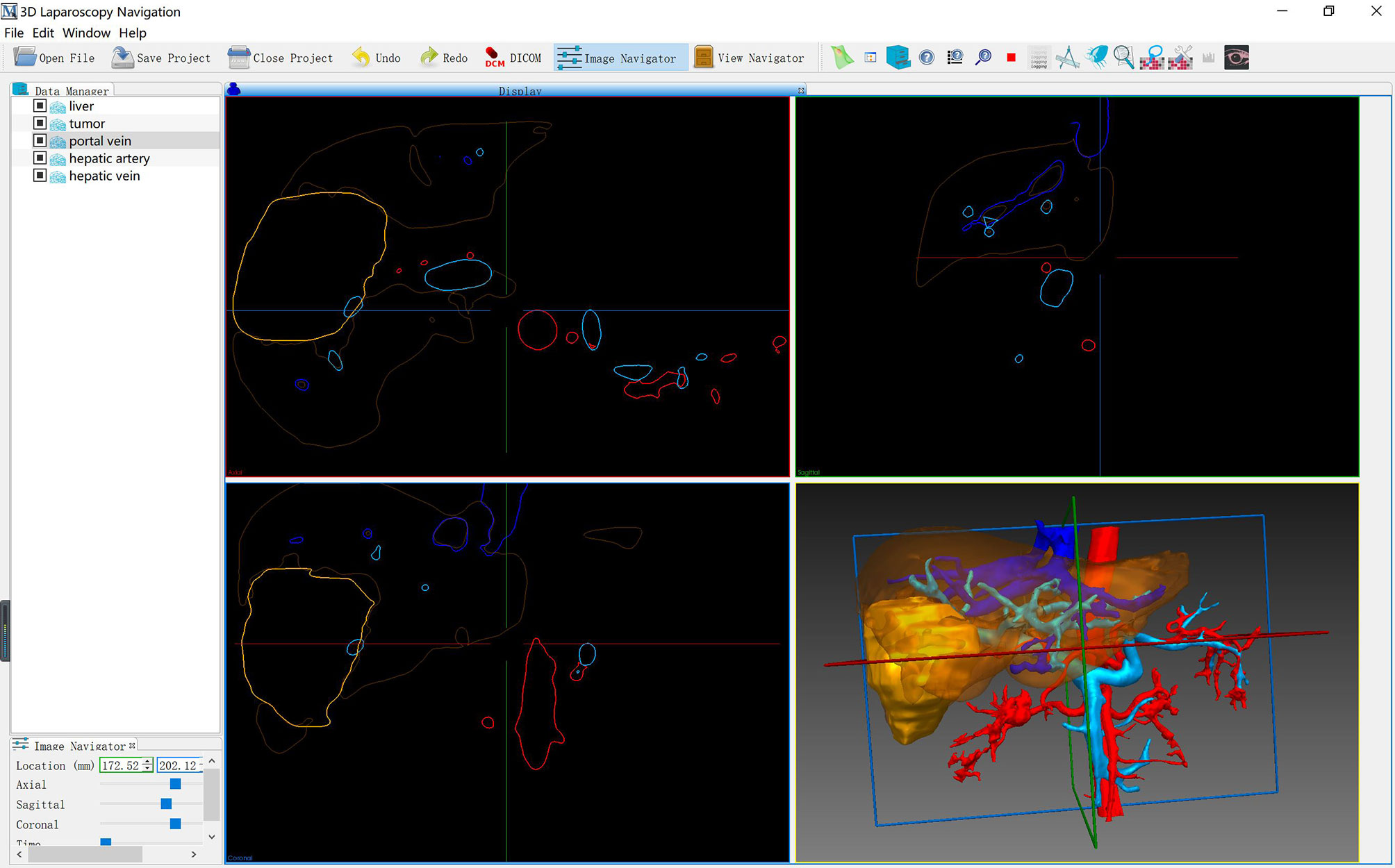The screenshot displays a detailed interface of a computer program named "3D Laparoscopic Navigation," identified in the upper left-hand corner next to a small "M" logo. The program's menu options, including File, Edit, Window, and Help, are visible beneath the title. The screen is divided into four quadrants, each showing different visualizations related to the "Portal Vane," the highlighted and open file on the left.

In the upper left quadrant, various segments of the Portal Vane are circled with primary colors—blue, red, and yellow—accompanied by green vertical and blue horizontal lines. The lower left quadrant features a similar color scheme, with objects circled and lines in green and red orientations. The lower right quadrant presents a 3D image of the Portal Vane, outlined with green and red lines, and surrounded by a blue box. Notably, a blue vane and a red vane are prominently highlighted, indicating their primary importance.

Across the panels, the colors and circles seem to represent different components, such as the liver, portal veins, hepatic arteries, and veins, which are checked off in a list within the program. This intricate layout is likely meant for use by surgeons or diagnosticians to navigate and understand complex anatomical structures during procedures.